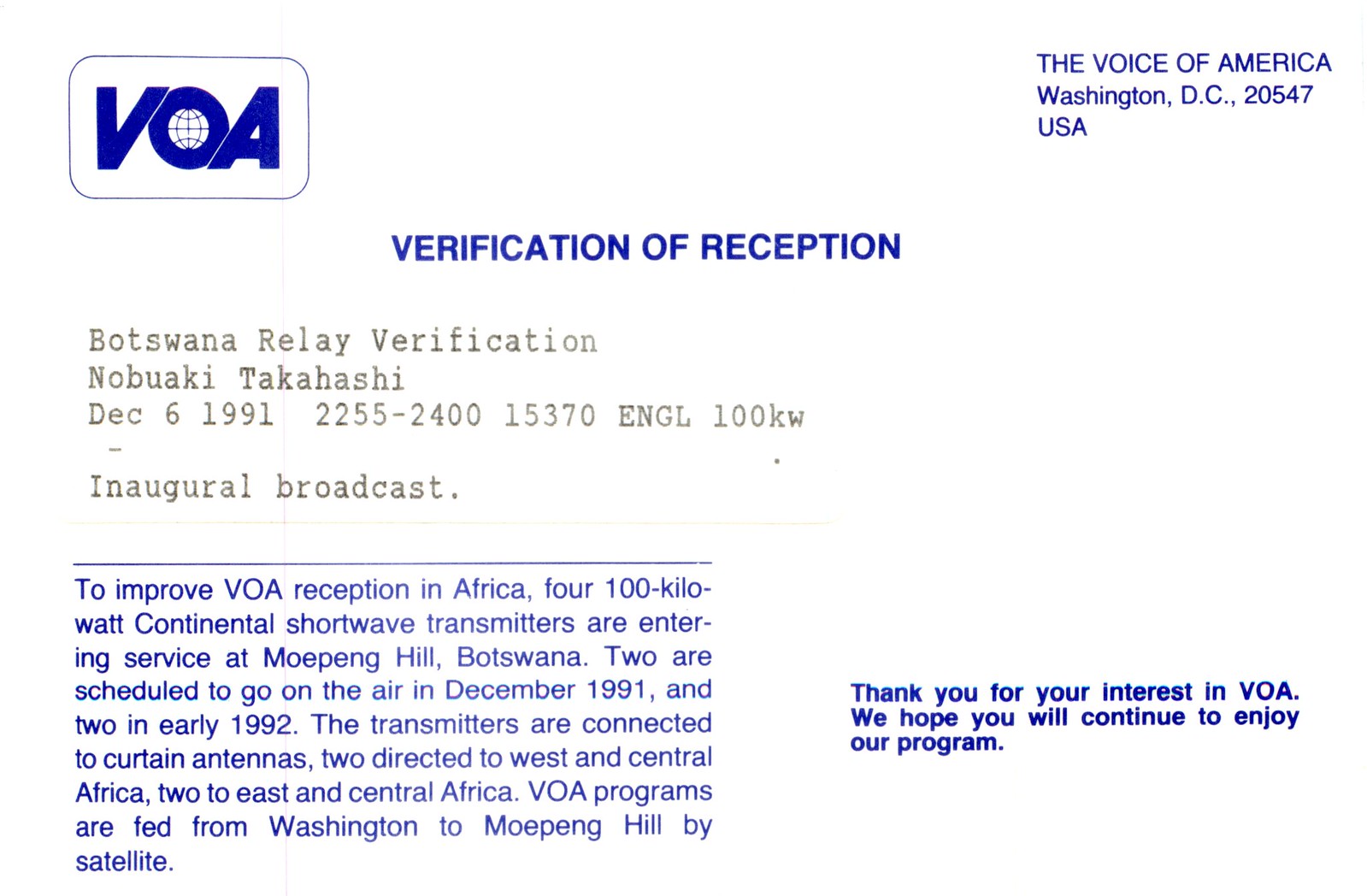The image displays a verification receipt from the Voice of America (VOA), specifically acknowledging a radio transmission. In the top left corner, the VOA logo is prominent, featuring "VOA" in blue capital letters with a globe centered within the letter "O," all enclosed within a rounded blue rectangle. The document is titled "Verification of Receipt" and is dated December 6, 1991. It confirms the Botswana relay verification for Nobuaki Takahashi, marking the inaugural broadcast of a 100-kilowatt shortwave transmitter at Maopeng Hill, Botswana, transmitted to 15370 ENGL from 22:55 to 24:00. The text details that four 100-kilowatt continental shortwave transmitters were introduced to enhance VOA reception in Africa, with two transmitters going on air in December 1991 and the remaining two in early 1992. These transmitters are connected to curtain antennas, designed for broadcasting to West, Central, East, and Central Africa. The VOA programs are fed by satellite from Washington to Maopeng Hill. The closing statement expresses gratitude for the listener's interest and hopes they continue enjoying the programs.